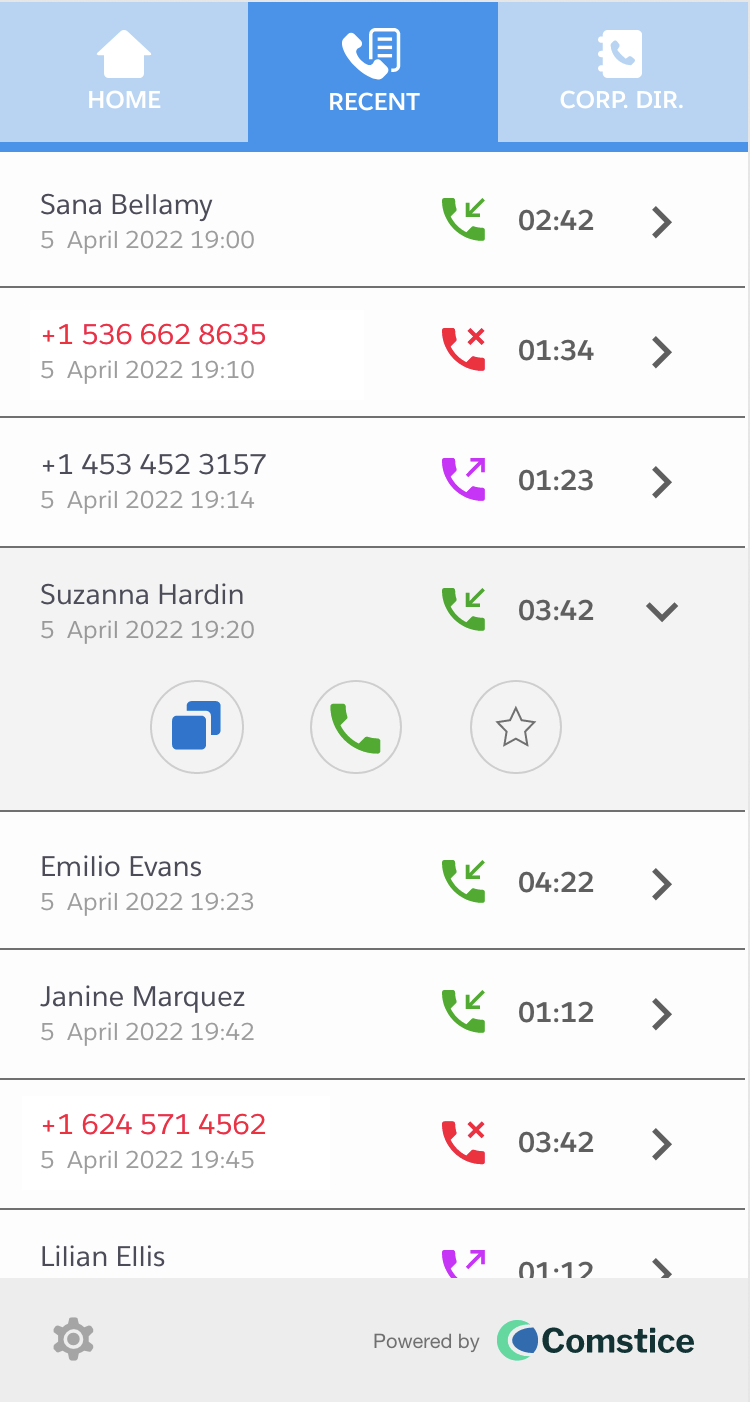**Detailed Caption:**

This is a mobile phone screenshot showcasing a call log. The top section of the screenshot features a blue band with three distinct blue squares: a dark blue square in the middle, flanked by lighter blues squares on each side, and a thin dark blue line running below them. Additional icons include a white home icon on the left, a recent icon depicting a phone in the center, and an icon that may signify "Copy" on the right.

Below this blue band, a list of names, phone numbers, dates, and call times is displayed. The bottom of the screen features a grey bar with a gear icon on the left side and the text "Powered by Comstas" on the right side.

The call log entries are as follows:

- **Sarah Bellamy**: April 5th, 2022 at 9:00 AM. The call, marked by a green phone icon, lasted for 2 minutes and 42 seconds.
- **Unidentified Red Number**: April 15th, 2022 at 7:10 PM. The call was not picked up, and it's marked with a duration of 1 minute and 54 seconds.
- **Unidentified Black Number**: April 15th, 2022 at 9:04 AM. The call, associated with a purple icon (possibly indicating an outgoing call), lasted for 1 minute and 23 seconds.
- **Susanna Harding**: April 5th, 2022 at 7:00 PM. This call, marked by a green phone icon, lasted for 3 minutes and 42 seconds, with additional blue copy, green phone, and star icons beneath it.
- **Emilia Evans**: April 5th, 2022 at 9:03 AM. This call lasted for 4 minutes and 22 seconds, indicated that they called the phone owner.
- **Janine Marquez**: April 5th, 2022 at 7:42 PM. The call lasted for 1 minute and 12 seconds, marked that they called the phone owner.
- **Another Unidentified Red Number**: A call that was not picked up at 7:46 PM on an unspecified date, having a confusing time duration of 3 minutes and 42 seconds.
- **Linnian Eilis**: Displayed with a purple icon and an incomplete call duration of approximately 12 seconds.

The screenshot appears to run out of space, cutting off part of the last entry.